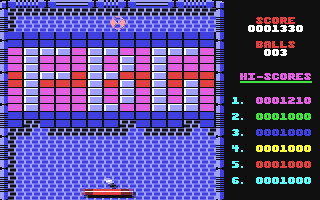The image depicts the classic arcade game Super Breakout. The game interface shows a vivid arrangement of colored bricks, with blue bricks at the top and bottom, pink and red bricks arranged in three separate lines in the middle, and grey bricks that spell out the letters "FBG." A red paddle at the bottom of the screen is positioned to deflect a floating steel ball. On the right side of the screen is a vertical black bar occupying a quarter of the screen. This bar contains several game statistics and labels: "Score" is written in red, followed by numbers "0 0 0 1 3 3 0." Below this, "Balls" are listed with "0-3" in white. The "High Scores" section is noted in magenta and underlined with green, displaying scores in baby blue font listed as 1, 2, 3, 4, 5, and 6 with the corresponding numbers in purple, green, red, yellow, red, and baby blue. The overall objective of the game is to use the paddle to keep the ball in play and break all the colored bricks.